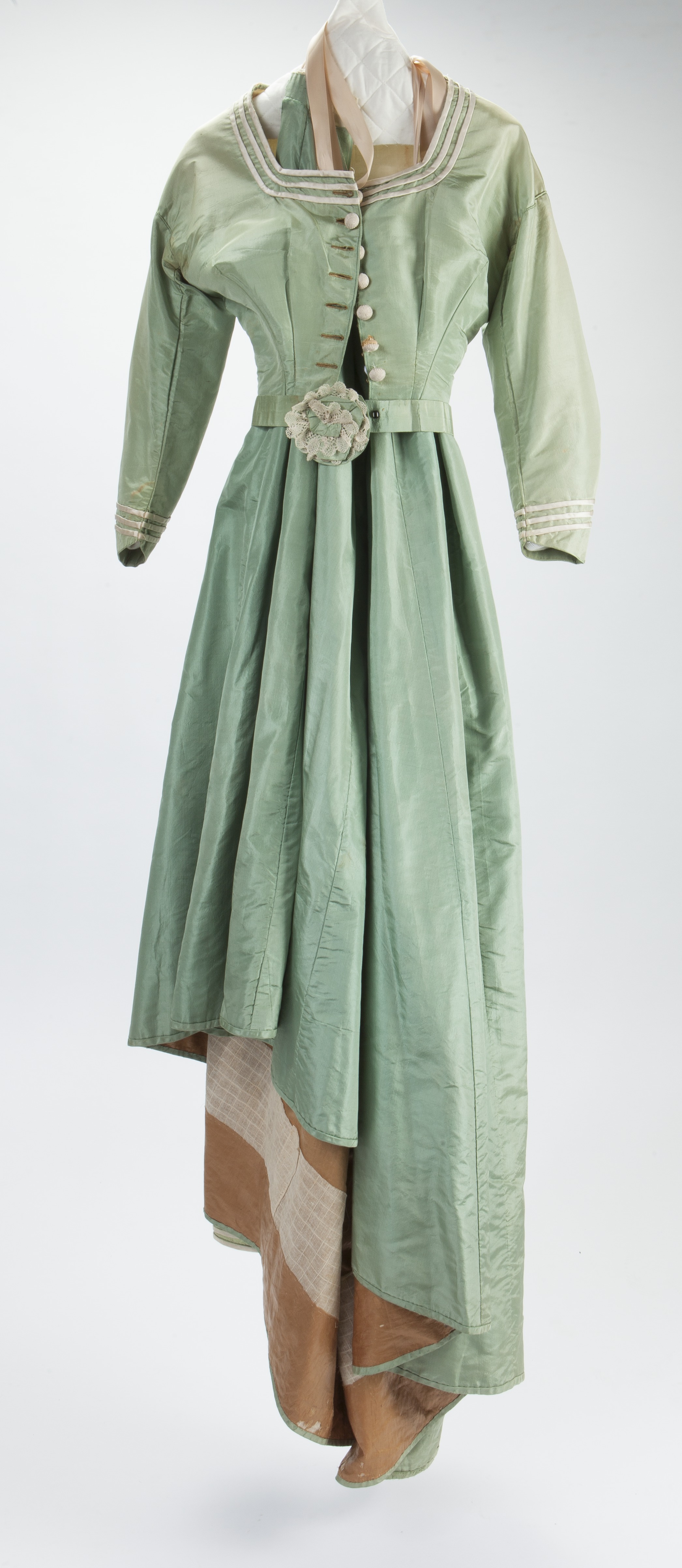This image features a traditional dress set against a light greenish background. The dress itself is a rich green color and showcases intricate details. It has a belt buckle adorned with a light green flower at the center. The long sleeves are accented with three distinctive white stripes around the wrist area. Running up the middle of the dress, a row of white buttons adds to its elegant charm. Additionally, three white line strips adorn the upper chest and neck area, providing a cohesive design element.

Underneath the dress, there appears to be a brown and white fabric layer. The base of the outfit extends into what seems to be a long-sleeved coat and skirt combination. The skirt portion is a shimmery green and is beautifully complemented by a brown and beige striped layer underneath, which gracefully reaches down to the floor. This detailed and ornate attire exemplifies traditional fashion, blending various textures and colors harmoniously.